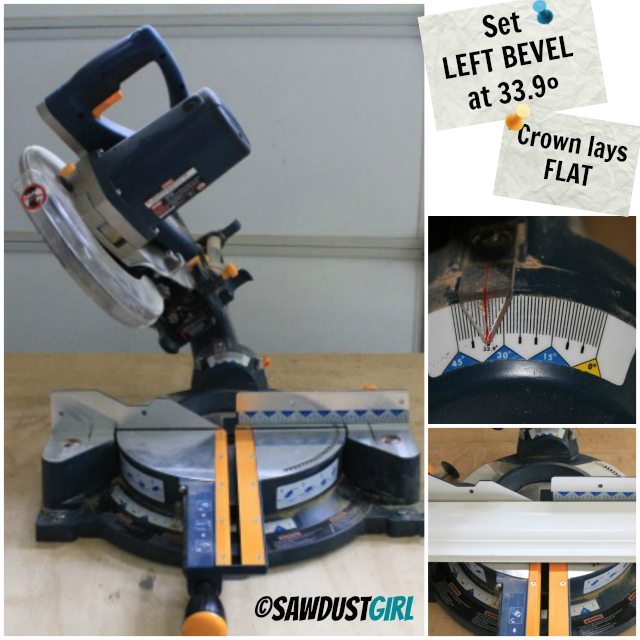The image features a detailed view of a miter saw, prominently positioned on the left side. The miter saw is blue with a metal base, and it includes a motor on the side and a handle on top which engages the blade. The base, anchored to a light wooden board, shows signs of frequent use with sawdust visible on it. A plastic guard on the saw ensures safety as the blade, with serrated edges, is brought down to make precise cuts at various angles.

In the upper right-hand corner of the image, two tacked signs provide specific operational instructions: "Set left bevel at 33.9 degrees" and "Crown lays flat." The signs are pinned with board pins and set against a white background. Below these instructions are two smaller, close-up photographs showcasing different parts of the saw, emphasizing its clean and well-maintained condition. One close-up reveals the detailed measuring stick on the saw, marked with various angles such as 45, 30, and 15 degrees. The saw also features an orange button to engage the blade and yellow handles for ease of use.

The bottom right corner of the overall image bears the label "Sawdust Girl," which could indicate either a brand name or the person who owns the saw. Additionally, a piece of white baseboard wood positioned on the saw base illustrates the setup for an impending cut, enhancing the instructional aspect of the image.